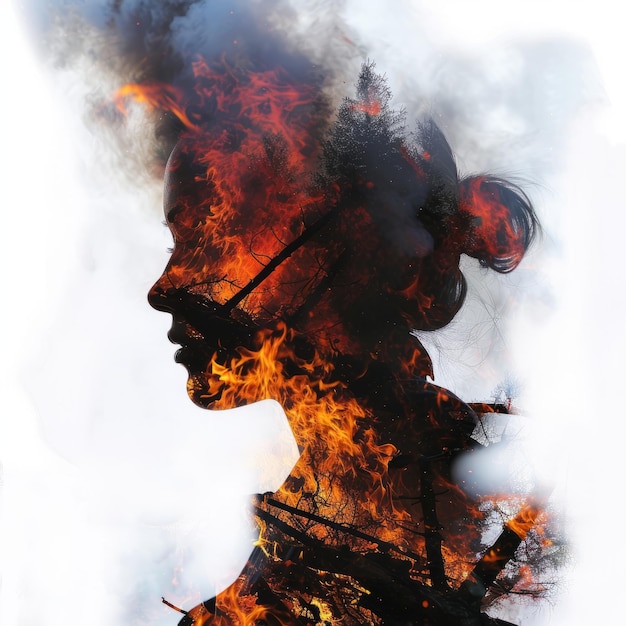This artistic digital image features a side profile silhouette of a woman with her hair pulled back into a bun, set against a stark white background. The woman's silhouette is intricately filled with a vivid depiction of a raging forest fire, characterized by deep red and orange hues of flames consuming trees and thick smoke rising around her. The smoke and flames blend seamlessly into her form, with flames emerging from her head and engulfing her neck and body, highlighting a sense of catastrophic devastation. The haunting scene within her silhouette powerfully contrasts against the simplicity of the surrounding white backdrop, emphasizing the intensity of the fiery chaos within. This evocative artwork seems to symbolize the destructive nature of widespread wildfires, perhaps drawing a parallel to real-life events such as those experienced in California.